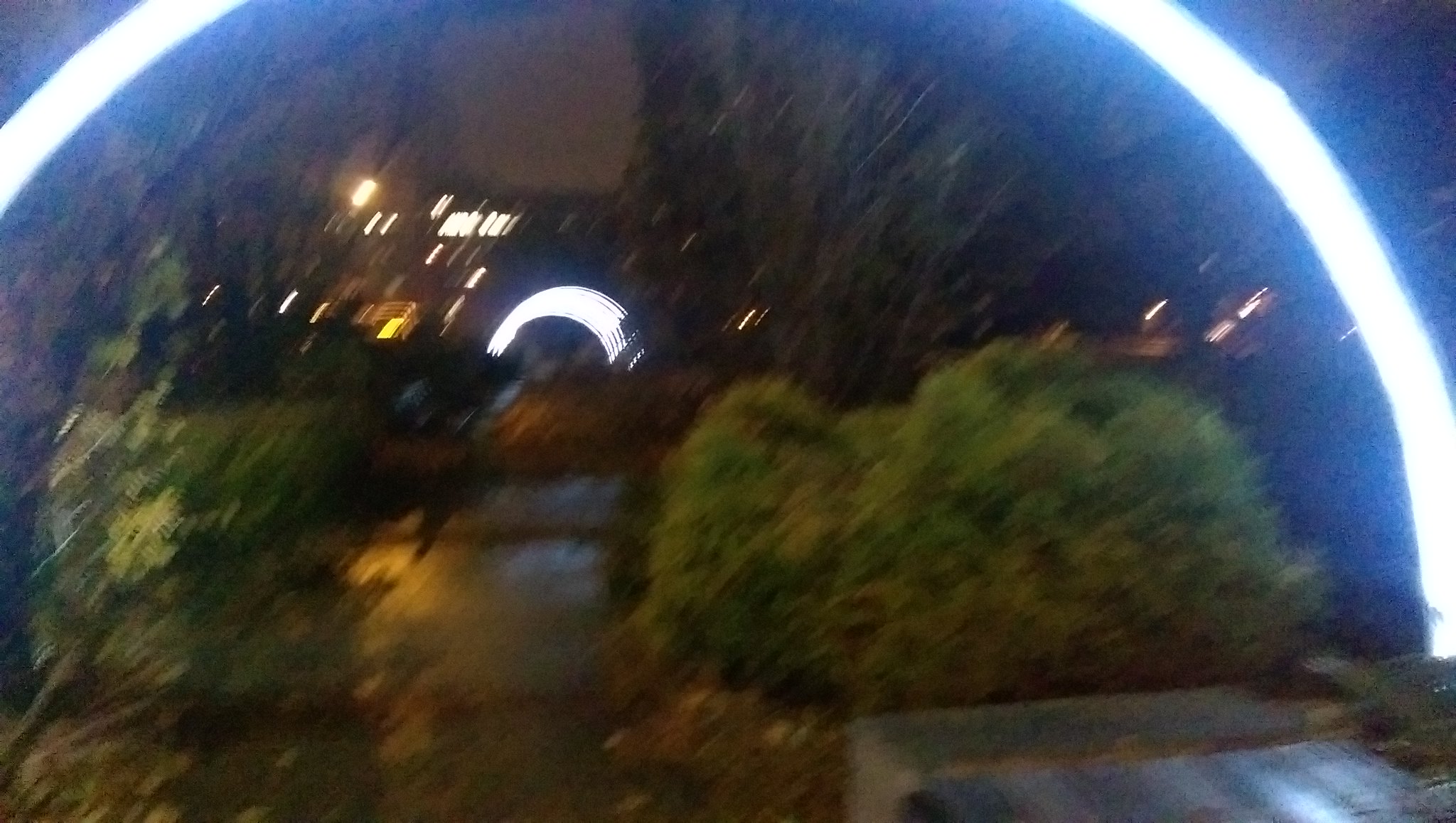The photo captures an enchanting outdoor scene featuring a radiant light installation that forms a halo-like arch. The luminous arch begins on the left side, moves to the front corner, and then gracefully disappears at the top of the image, only to reappear on the right side. Multiple similar light arches can be seen stretching ahead in a mesmerizing row, creating a tunnel-like effect. The walkway beneath these glowing arches is flanked by lush green shrubs and trees. A wooden crate is positioned at the bottom right of the photo, adding a rustic touch to the scene. Brown foliage sporadically grows between the cracks of the pathway, adding to the natural ambiance of this beautifully illuminated passageway.